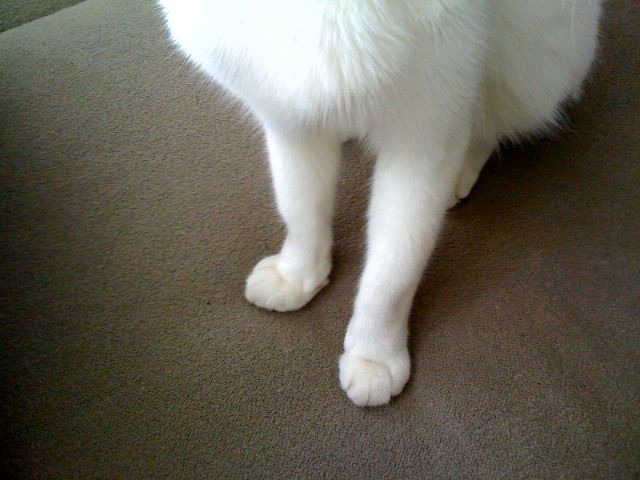In the photograph, the shooter captures a downward view from their seated position, focusing on a white long-haired cat positioned on what appears to be a gray, fluffy, cotton-polyester armrest of a couch or chair. The cat is poised on all fours, facing the camera, with the shot specifically featuring its chest, front legs, and a portion of the back end. Illuminated by a light source behind the camera, the cat's thick, luxurious white chest fur contrasts with its smaller, delicate front paws which are pressed into the soft fabric. The image also reveals the backside of the cat, partially obscured in shadow but showing one haunch and a few toes of the back foot, indicating the cat is seated comfortably with a back leg tucked underneath. The absence of the head and tail draws attention to the texture and placement of the cat's fur and the softness of its surroundings.